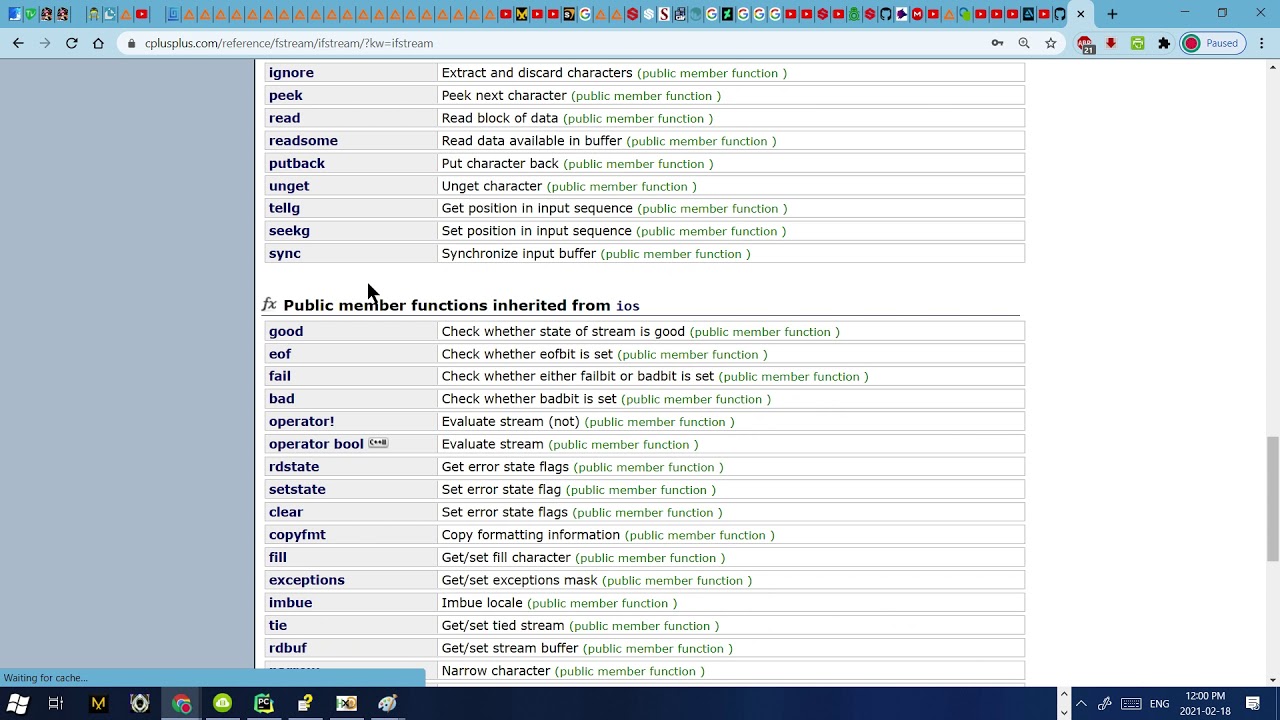The image is a detailed screenshot of an online page formatted in a wide rectangular shape. At the top, there's a pale blue border filled with various icons spanning its length. Beneath this, an even paler blue border contains a white space displaying a URL in black text, flanked by icons on both the left and right sides.

In the middle section of the image, several horizontal lines represent lists, each aligned with gray empty space to the left and white empty space to the right. These lists appear to detail various options or actions. 

Starting from the top left and extending vertically in the center, there is a list with the following labels: "ignore", "peek", "read", "read some", "put back", "unget", "tell G", "seek G", and "sync". Each of these items has a corresponding description to its right:
- "ignore" - Extract and discard characters (public member function)
- "peek" - [Description] (public member function)
- "read" - [Description] (public member function)
- "read some" - [Description] (public member function)
- "put back" - [Description] (public member function)
- "unget" - [Description] (public member function)
- "tell G" - [Description] (public member function)
- "seek G" - [Description] (public member function)
- "sync" - [Description] (public member function)

Each description is in black text, and every description ends with the phrase "(public member function)" in green text.

Beneath this section, another list bears the heading "FX, public member functions inherited from IOS". This list aligns directly under the "sync" label from the previous list. The items listed from top to bottom include: "good", "EOF", "fail", "bad", "operator!", "operator bool", "rdstate", "setstate", "clear", "copyfmt", "fill", "exceptions", "imbue", "tie", and "rdbuf". Similar to the first list, each item in this list also has a corresponding description to its right, with black text descriptions ending with "(public member function)" in green text.

At the bottom of the screen, there is a dark border featuring several icons on both the left and right sides. The Windows icon is prominently displayed in the lower left corner, along with other icons positioned to the right of it.